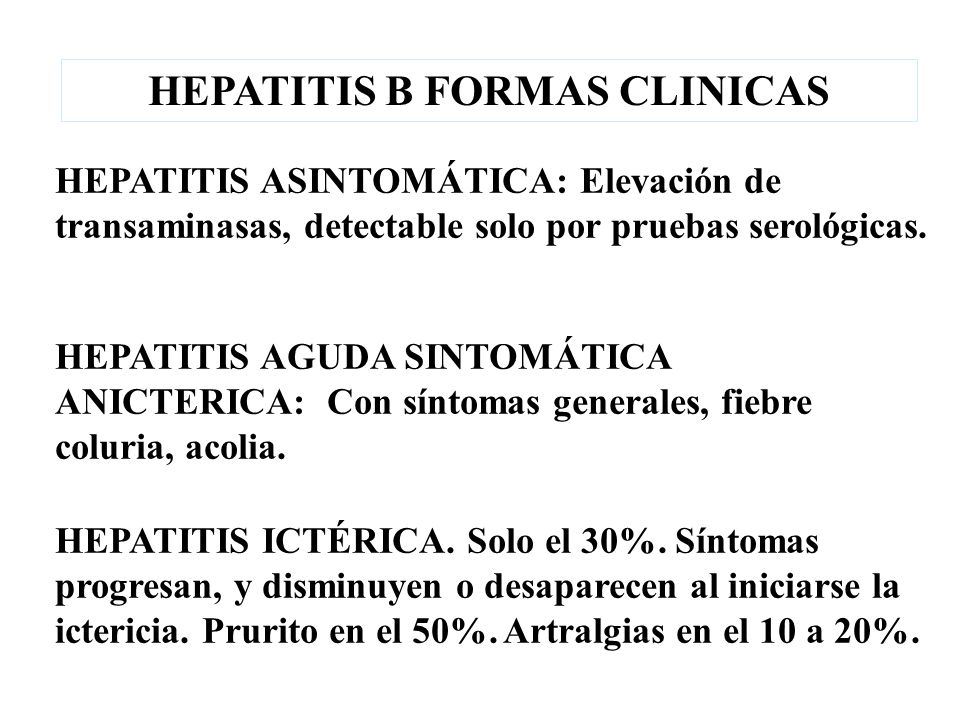The image presents an informational slide or poster with a white background and black text. At the top, there is a centered title in all caps with a thin light blue rectangular border around it, reading "HEPATITIS B FORMUS CLINICUS." Below this main heading, the information is left-aligned detailing various clinical forms of Hepatitis B, written in Spanish. The first section, titled "Hepatitis Asymptomatica," describes the condition as detectable only by serological tests, stating "Elevación de transaminasas detectable solo por pruebas serológicas."

Further down, in the center of the image, another heading reads "Hepatitis Aguda Asymptomatica Anecterica," noting symptoms like general malaise, fever, dark urine (choluria), and pale stools (acolia).

The final section, concerning "Hepatitis Ecterica," mentions that 30% of cases progress or remit with the onset of jaundice, with pruritus occurring in 50% of cases and arthralgia in 10-20%.

In summary, this is a detailed, Spanish-language informational slide on Hepatitis B with sections describing asymptomatic and symptomatic forms, specific symptoms, and statistics on symptom prevalence.